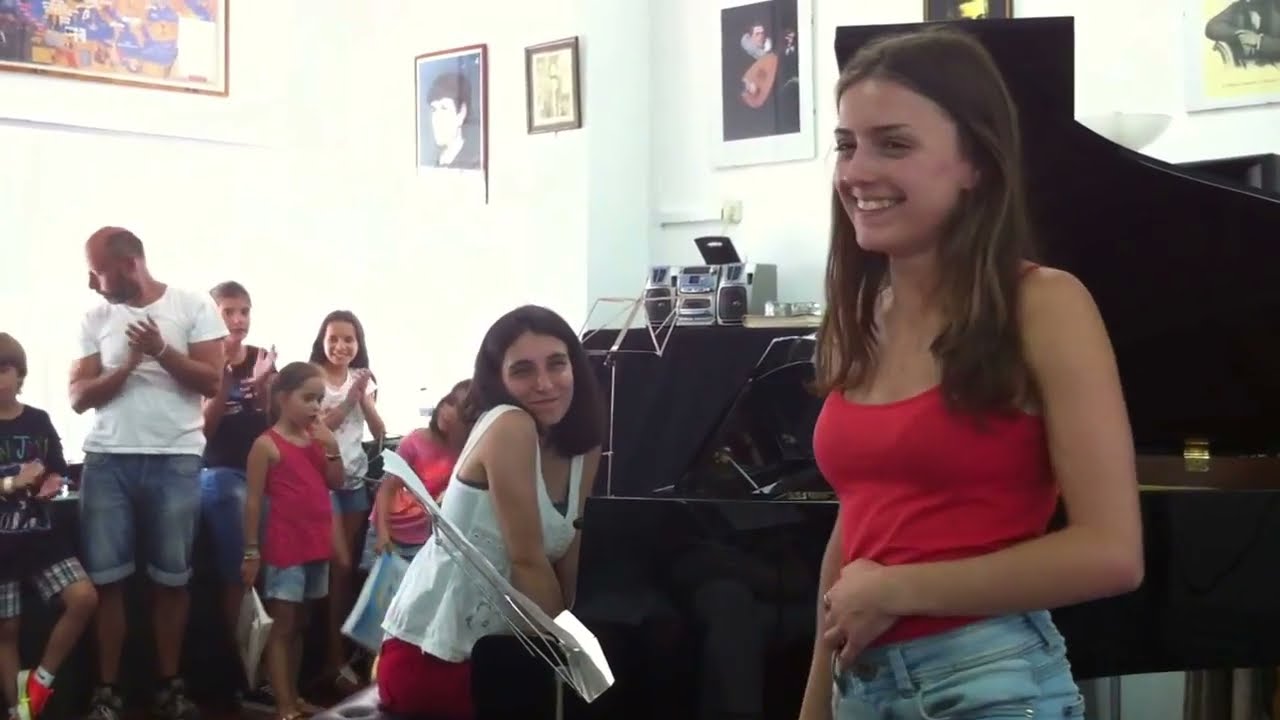The image is taken indoors, showing a lively gathering of children and two adults in a room with white walls adorned with various paintings and photos. The focus is on two pre-teen girls standing in front of a black grand piano. The girl in the foreground has medium-length, slightly wavy brown hair cascading over her shoulder. She wears a red tank top and blue jeans, smiling broadly and looking towards the left. Her right arm hangs down while her left hand rests on her stomach. Next to her, another girl, with shoulder-length dark brown hair, leans against the piano. She is dressed in a white tank top and red pants, also smiling.

Several other children, along with a male adult in a white t-shirt and blue jean shorts, are gathered around them. The man is clapping, glancing down at a boy to his right. The children, numbering four girls and two boys, join in the applause, adding to the sense of cheerfulness and celebration in the room. In the background, a grayish-silver boombox stereo and various portraits, including one of a person playing a Spanish acoustic guitar, further detail the setting. The scene suggests a musical performance or recital, where the group is applauding, possibly in admiration of the girl's recent performance.